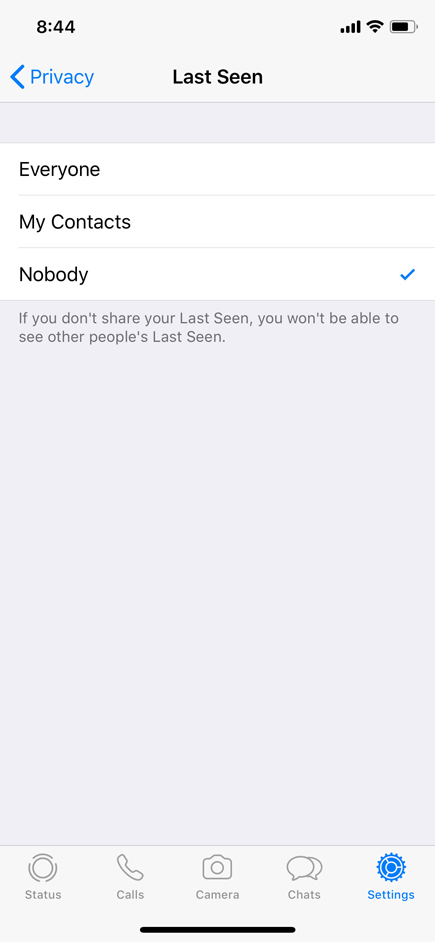### Detailed Caption for the Image:

This vertically-oriented image, likely captured from a smartphone screen, primarily features a light gray backdrop with black text and select blue elements for emphasis. At the very top, the current time is displayed as "8:44" in the right corner. Adjacent to the time display, indicators for signal strength, Wi-Fi connectivity, and battery life are positioned on the rightmost side of the screen.

Directly under this top section lies a slightly darker gray band, beneath which the word "Privacy" is prominently displayed in blue text with a blue left-pointing arrow adjacent to it. In line with this, but slightly to the right and centered at the top section's middle, the text "Last Seen" is visible.

The screen is divided into sections below the gray band. The first section lists three options for setting visibility preferences for "Last Seen" status, all aligned flush to the left:
1. **Everyone**
2. **My Contacts**
3. **Nobody** - this line has a blue checkmark to its right, indicating it is the currently selected option.

These selection options are set against a white background and are separated by thin light gray lines.

Beneath these options is a nearly square-shaped area, slightly wider than it is tall. It is mostly empty except for a message at the top in darker gray text: "If you don't share your last seen, you won't be able to see other people's last seen."

Finally, at the bottom of the screen, there is a lighter gray navigation bar that accommodates five icons from left to right:
1. **Status** - with a circular icon constructed with broken lines.
2. **Calls** - represented by a telephone receiver icon.
3. **Camera** - denoted with a sketch of a camera.
4. **Chats** - indicated with a chat bubble icon.
5. **Settings** - both the text and its associated gear-like icon are in blue and white, located at the far right of the bottom navigation bar.

Each icon is labeled and serves as options for different functionalities within the app.